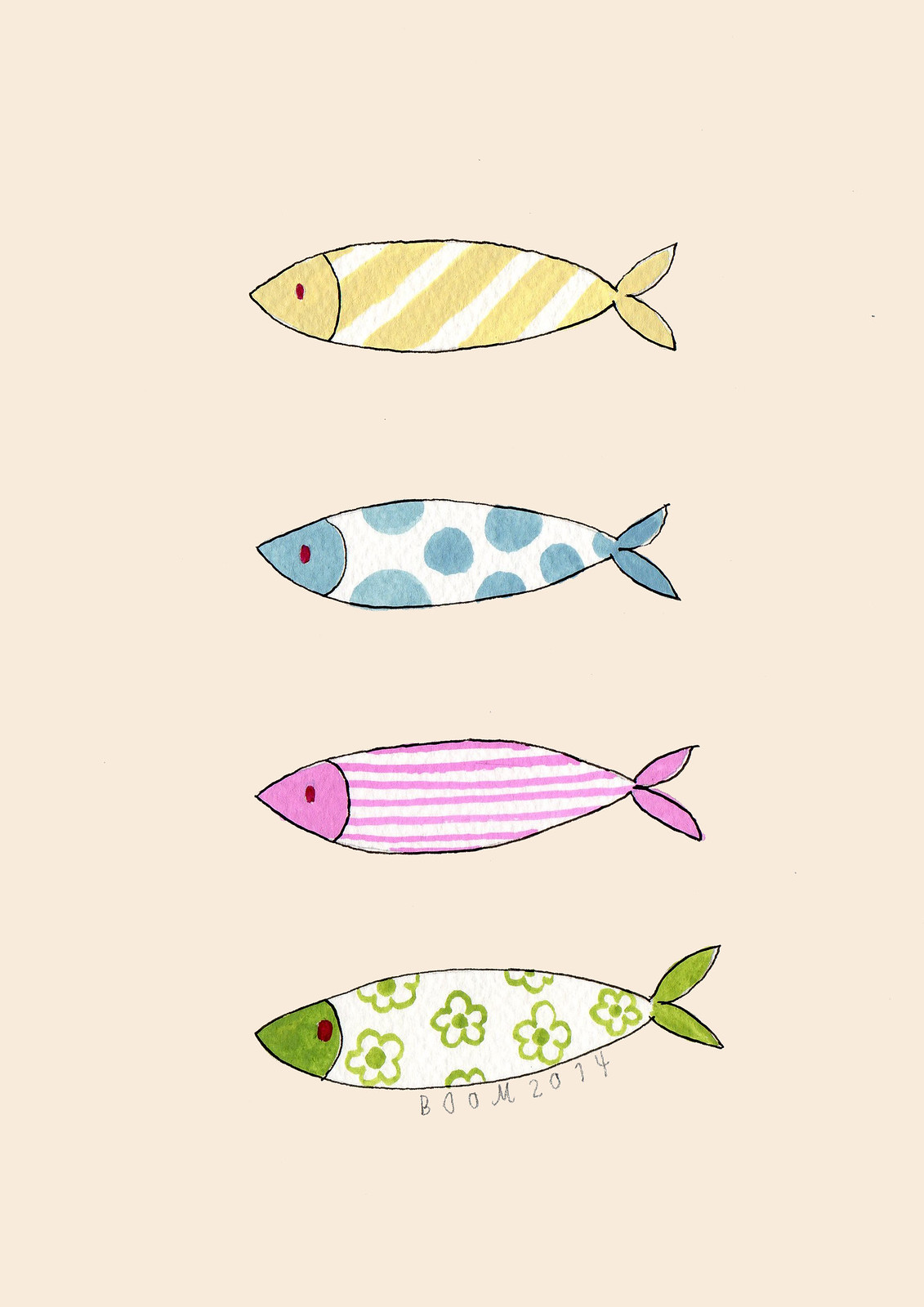This artwork features four intricately designed and brightly colored fish set against a plain beige background. Each fish is drawn with a distinctive combination of patterns and hues, and all of them have a characteristic red eye.

1. The top fish showcases a yellow head, occasionally described as orange or peach, adorned with maroon or red eye. Its body features alternating diagonal stripes of yellow and white, culminating in a yellow tail fin.
2. The second fish boasts a blue head with a red eye. It has a white body decorated with blue polka dots, some of which are positioned at the top and bottom edges, and a blue tail fin.
3. The third fish exhibits a pink head and a red eye. Its body is marked by horizontal pink and white stripes, and it ends with a pink tail fin.
4. The bottom fish has a green head with a red eye. The white body is embellished with green flower prints outlined in green with white interiors, and it finishes with a green tail fin. 

An artist’s signature, "Boom 2014," is inscribed beneath the green fish, indicating the creator of this vivid and imaginative illustration.